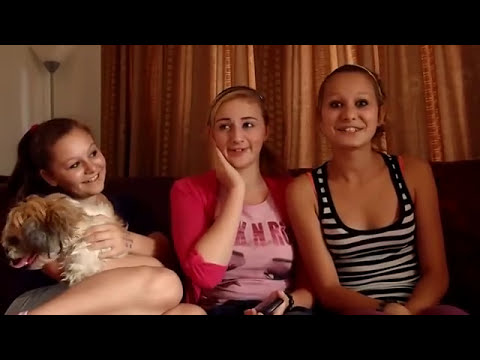In this vibrant photo, three young girls, possibly teenagers, are seated on a dark, perhaps black, sofa. Behind them, rich brown curtains drape down vertically, and a torch lamp stands in the corner of the room. The girl on the left, who has brown hair, is smiling warmly as she cradles a small, shaggy brown and white dog atop her tucked-up legs. In the center, the girl with either blonde or red hair is wearing a red and pink sweatshirt with visible lettering reading "K" and "G." She holds her right hand to her chin, seemingly in a playful, "oh my" gesture, while smiling and glancing towards the right. The girl on the right, dressed in a sleeveless black and white striped tank top, leans forward slightly with an excited expression. She has a bandana in her hair and positions her hands in front of her. All three girls are radiating happiness and excitement, captured in a perfect moment of youthful joy.